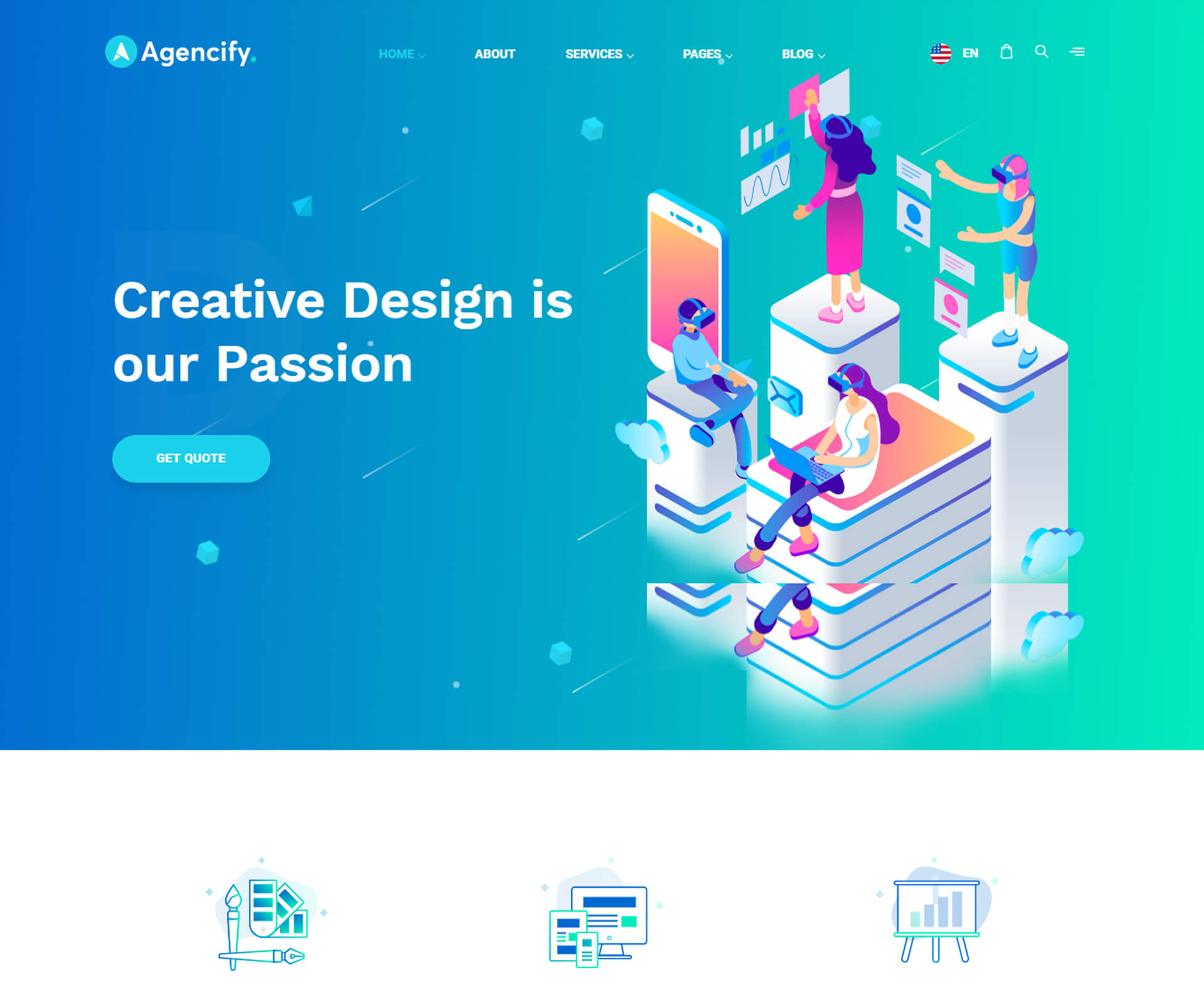The image is a detailed brochure from "Agent 5," featuring their distinctive logo—a teal circle with the tip of an arrow, resembling a triangle with a rounded base. The background transitions smoothly from dark blue to a green-blue and finally to green. The navigation menu at the top includes sections labeled "Home," "About," "Services," "Pages," and "Blog," alongside an American flag icon for English language selection. The "Home" section is highlighted, indicating it is the current page.

The main tagline, "Creative design is our passion," is prominently displayed, accompanied by a teal button labeled "Get Quote." To the right, four individuals are engaged in virtual reality activities, each standing or sitting on unique columns. 

- The boy, dressed in a blue sweater and jeans, stands on one of the columns.
- A girl with long black hair, wearing a pink dress with matching pink shoes and white socks, stands on another column.
- Another girl, in a matching top and shorts paired with blue shoes and white socks, occupies a third column.
- Finally, a girl seated on a column wears a dress and leggings, along with blue socks and pink shoes.

Below this scene, there are various symbols: two depicting the lantern from the Statue of Liberty, a dry erase board, and another dry erase board featuring a bar graph.